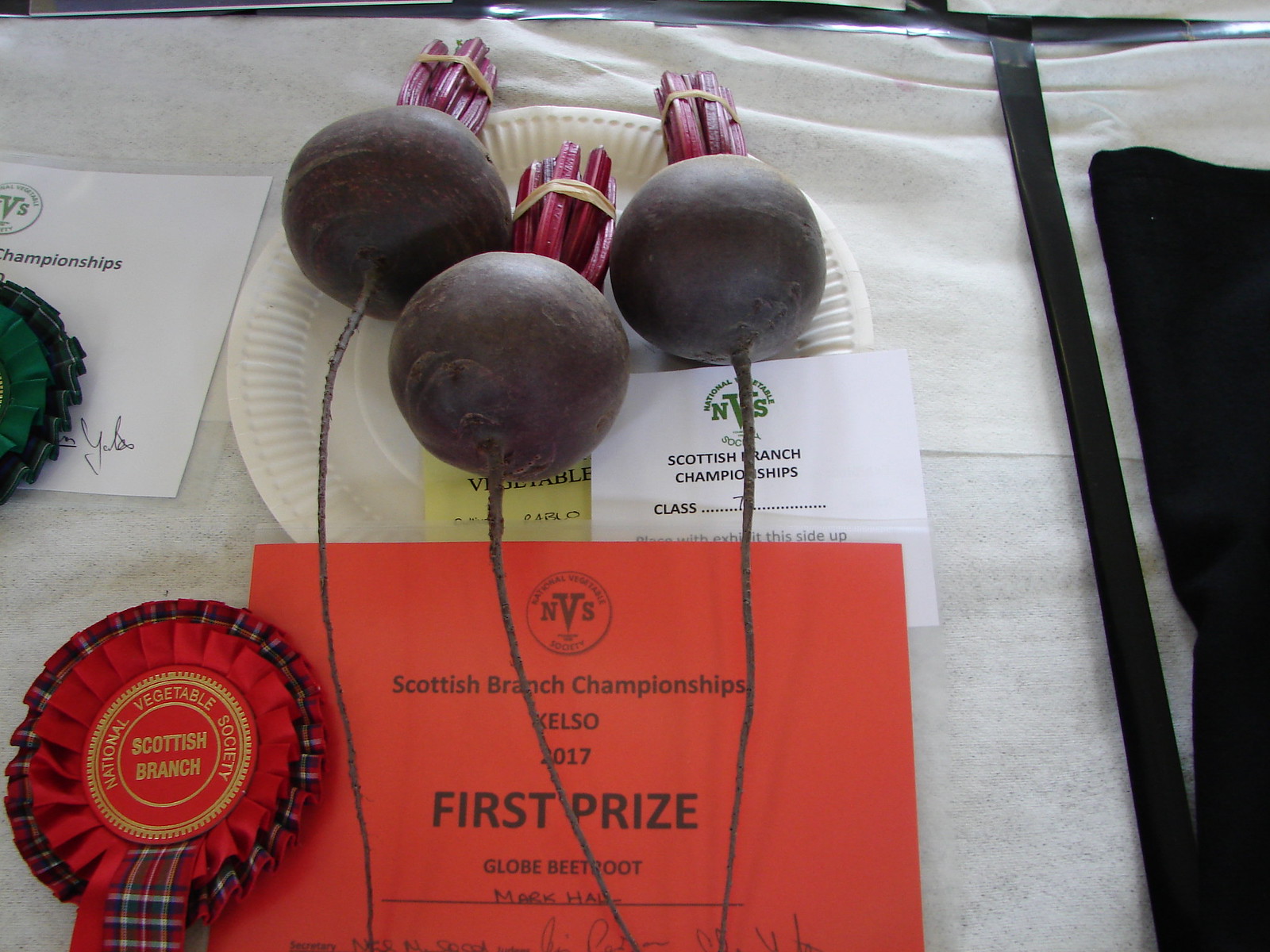In the photograph, a paper plate displayed prominently on a large table holds three prize-winning globe beetroots, each firmly bound with a rubber band. These beetroots, resembling round cannonballs with burgundy-colored stalks, dominate the center of the image. An orange certificate beneath the plate details the accolade: "National Vegetable Society, Scottish Branch Championships, Kelso 2017, First Prize Globe Beetroot.” Adjacent to the certificate, a red ribbon bearing the inscription “National Vegetable Society, Scottish Branch” adds a touch of prestige. The background colors include black, white, off-white, purple, brown, yellow, green, orange, red, and gold, creating a vibrant setting that looks reminiscent of a county fair vegetable award ceremony.